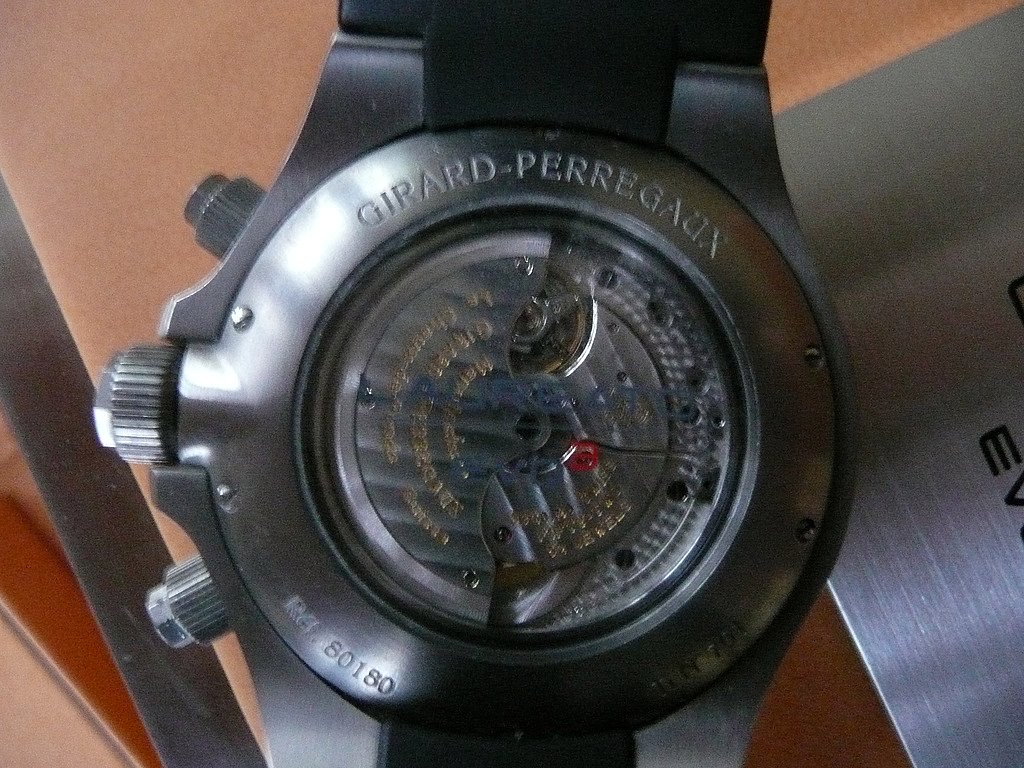The close-up color photograph captures the intricate details of the bottom of a wristwatch. The watch features a matte chrome-colored round body with a refined matte finish. At the center of the watch's underside, the inner workings are visible through a see-through screen, showcasing a fascinating display of mechanical craftsmanship. Gold-etched inscriptions surround the display, likely indicating the place of manufacture and the company name.

Encircling the outer rim of the bottom casing, the words "Girard-Paraguay" are prominently inscribed. Below these inscriptions, a reference number is marked. The side of the watch exhibits three buttons: a primary turning knob and two secondary pusher buttons, enhancing the watch's functionality.

The watch is equipped with a black strap, which appears to be made of either rubber or leather, blending seamlessly with the watch's design. Directly adjacent to the strap, a brushed metal plate with black characters is partially discernible, though most of the text remains unreadable. This plate also matches the watch's brushed metal finish.

The background underneath the watch consists of a blend of beige, orange, and hints of dark brown, providing a contrasting backdrop that highlights the watch's sophisticated details.